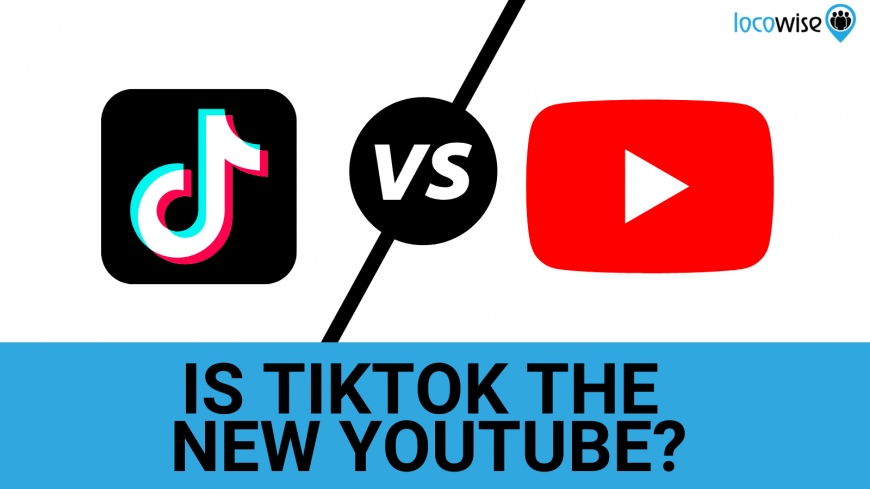This image is a cropped desktop screenshot with extensive white space occupying approximately three-fourths of the area. The specific web address, browser type, and operating system are not visible. In the top right corner, the word "LOCO WISE" is displayed as a single entity; "LOCO" is in pale blue, while "WISE" is in black. Accompanying this text, there is a blue location map pin containing three people icons.

Below this, there is a prominent black square with a white music note resembling a semi-3D effect, recognizable as the TikTok icon. Adjacent to it, a black circle with the word "versus" written in white sits between a black slash and backslash. Next to this element is a red square featuring a white triangle pointed to the right, representing the YouTube icon. 

At the bottom of the image, a medium blue rectangle contains the text, "Is TikTok the new YouTube?" The overall composition and the elements present suggest that the image is likely designed as an ad or clickbait graphic, presumably linked to an article discussing the comparison between TikTok and YouTube.